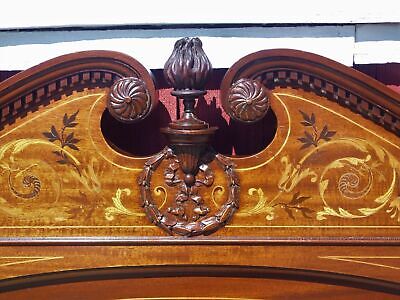This photo captures the ornate wooden carving that adorns the top of a vintage furniture piece, likely an armoire, headboard, or dresser. The dark-stained wood features intricate scroll designs on the left and right, curling elegantly like seashells. The central section showcases an elaborate torch-like structure that rises from the center, crowned by what appears to be a bird. The carvings extend to include delicate vine and leaf motifs, with some areas highlighted by lighter, yellowish inlay. The entire piece is richly decorated with filigree and floral patterns, giving it an antique and crafted feel. The image hints at the sun shining down, illuminating the carvings and accentuating the contrast between the dark wood and the lighter carved elements, creating an impression of an elegant, vintage masterpiece.